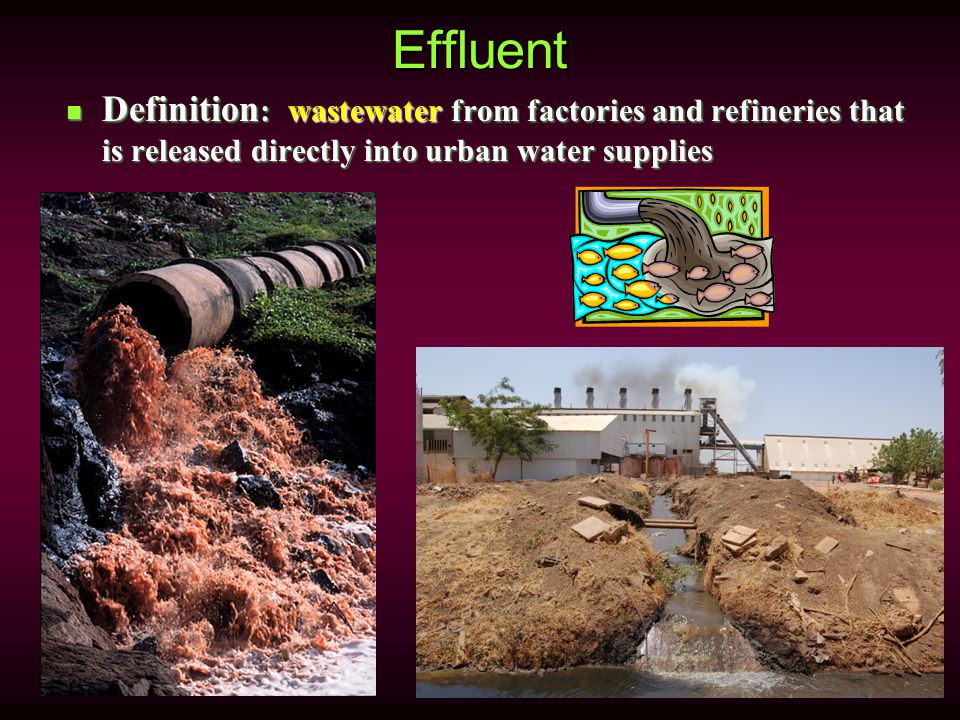The image depicts a slide from a PowerPoint presentation with a dark magenta background that fades to almost black at the edges. At the top of the slide, the word "Effluent" is prominently displayed in light green neon text. Below it is a small neon green bullet point followed by white text that reads "Definition:". The definition itself is highlighted in yellow and states "wastewater," followed by white text explaining it as "from factories and refineries that is released directly into urban water supplies."

On the left side of the slide, there is a photograph of a large concrete pipe partially seated on green grass, releasing a rapid flow of murky, brown water into an adjacent water stream. On the right side, another image shows a factory with smokestacks emitting smoke. Below the factory, pipelines also discharge contaminated water into a nearby river. Both images illustrate the pollution impacting urban water supplies. The stark visuals and vivid text colors contrast sharply with the dark, ominous background, emphasizing the serious environmental issue being presented.